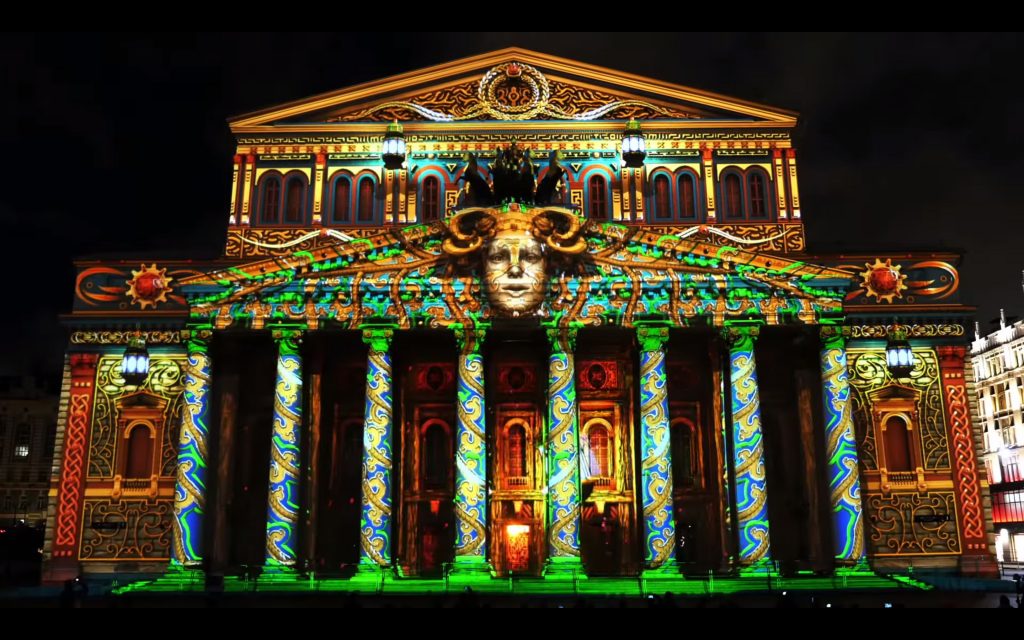The image depicts the front of the Bolshoi Ballet building in Moscow, captured at night during the Moscow Circle of Light Festival. The entire facade of the building is illuminated with an HD projection, transforming its appearance. The structure, resembling a grand courthouse with its numerous tall columns, showcases intricate details through vivid colors and designs. Each of the eight columns is highlighted with blue and gold trim and accented by green lights at the top and bottom. Ivy in hues of brown and green is projected to appear as if it's creeping up the columns.

At the center of the overhang, a prominent projection of a court jester’s face looks directly at the viewer. The jester’s face is primarily white with accents of orange and yellow on its nose, between the eyes, and on the cheeks. It sports a gold floppy hat with curved corners resembling horns that twist outwards and then inwards. Surrounding this whimsical face are multicolored flourishes and script fonts, adding to the festive atmosphere. Above, an additional floor features arched windows and a pitched roof culminating in a pointed top with concentric rings just below the peak. The background of the photograph is pitch black, emphasizing the striking luminescence of the building’s ornate facade.